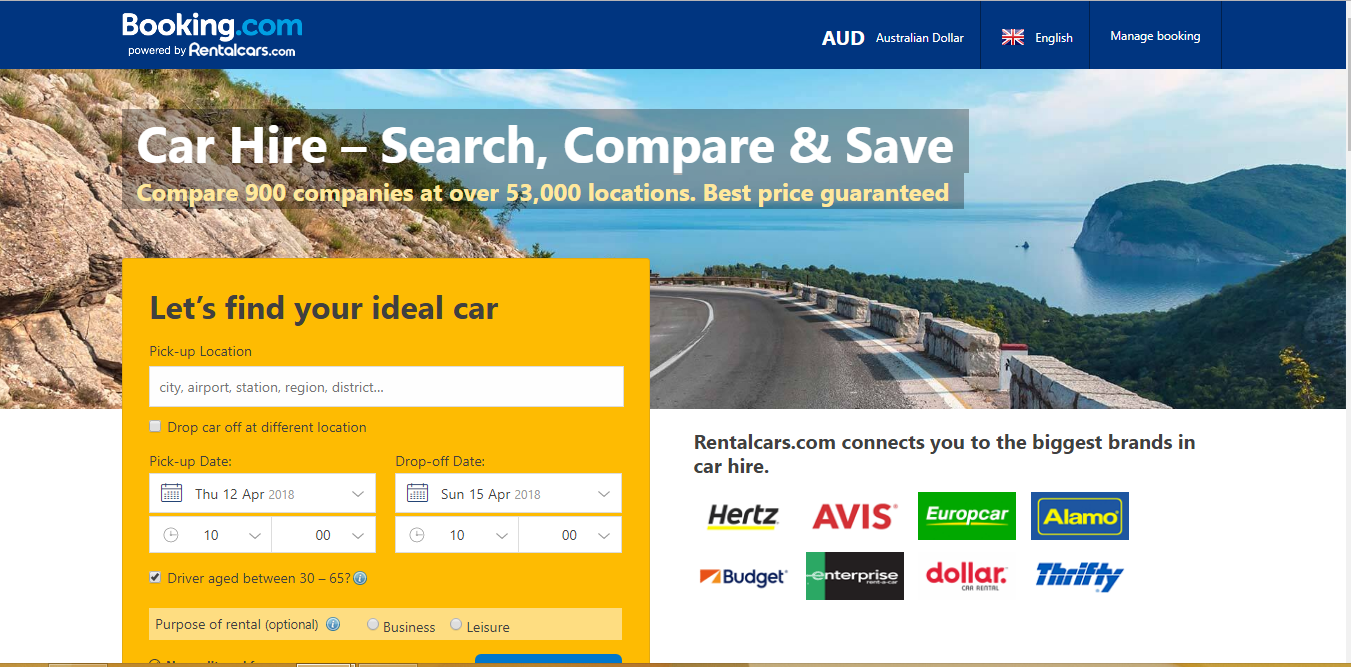A cropped screenshot of the Booking.com homepage showcases the platform's car hire section. At the top left, the Booking.com logo is prominently displayed, with "Powered by Rentalcars.com" subtly positioned underneath in small white letters. To the right of the logo, "AUD" appears twice, with the first in large white letters indicating the currency setting to Australian dollars, followed by a smaller "AUD." A British flag is situated alongside the word "English," also in small white letters. On the far right, the phrase "Manage Booking" appears in small white text.

Below the blue header, the prominent background features a captivating image of a road winding through mountains beside a sea. Overlaying this scenic backdrop is bold white text that reads, "Car Hire, Search, Compare and Save." Beneath it, in small yellow letters, the text declares, "Compare 900 companies at over 53,000 locations. Best prices guaranteed."

Towards the bottom left of the image, a large yellow box invites users to find their ideal car with the text "Let's find your ideal car" in large black font. Below this prompt, a text box is provided for the "Pick-up location," along with an option to choose a different drop-off location. Further down, two sections allow users to select "Pick-up date" on the left and "Drop-off date" on the right. The bottom right corner of the page highlights that Rentalcars.com connects users to the biggest brands in car hire, accompanied by the logos of eight major companies: Hertz, Avis, Europcar, Alamo, Budget, Enterprise, Dollar, and Thrifty.